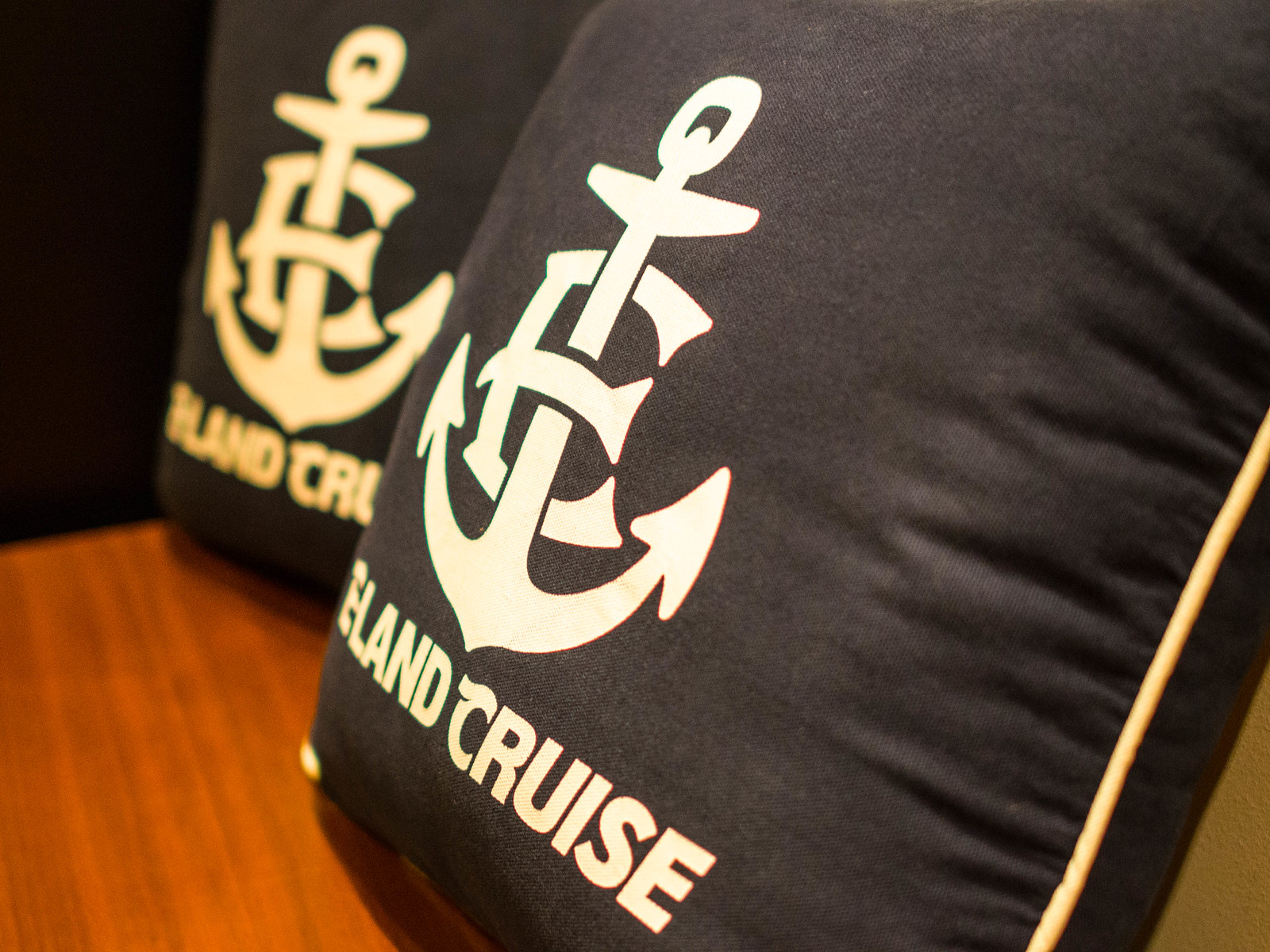The image features two decorative gray pillows with a light beige ribbing around the seams, positioned at a diagonal angle and partially cut off. Both pillows display a prominent anchor design on the front, intertwined with an ornate letter "E" such that parts of the E overlap and seem to hold the anchor. Below this emblem, the text "Island Cruise" is visible. The pillows rest on an orangey-brown table, positioned next to each other, with one pillow more towards the upper left and slightly out of focus. Behind the pillows, on the upper left, the background appears dark black.